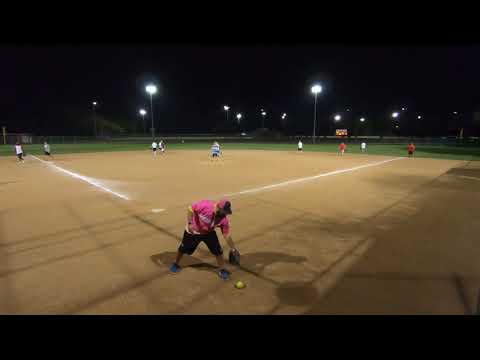Under the night sky, a lively baseball game unfolds on an outdoor field illuminated by numerous light poles scattered throughout. The image, taken from behind home base, prominently features a player in the foreground bending down to pick up a highlighter-yellow softball with their glove. This player is distinguished by their unique attire: a bright pink jersey with subtle yellow accents around the sleeves and collar, paired with black shorts, blue sneakers, and a black-and-pink hat.

In the background, the field's characteristic light brown clay playing area is clearly defined, with white chalk lines marking the boundaries and bases. Beyond the clay infield lies a lush green outfield where several players, although blurry due to the distance, stand in their positions. They are dressed in a mix of red, white, and black casual clothing, adding to the vibrant scene. A fence line can be seen far in the distance, enclosing the bustling activity of the game.